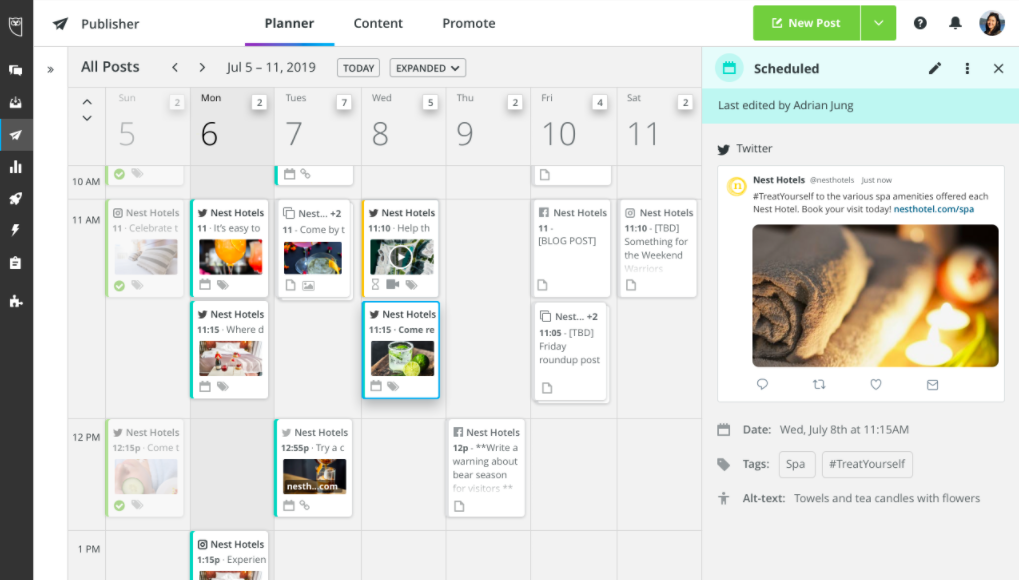The image is a screenshot of a website interface with a user-friendly design for managing and organizing content. 

On the left, a vertical black strip features several icons, each representing different functions. At the top of the page, there are tabs labeled "Publisher," "Planner," "Content," and "Promote." Below these tabs, a green bar prominently displays a button labeled "New Post" with a drop-down arrow for additional options. 

A profile picture of a woman is visible near the upper right corner, adjacent to a notification bell icon and a circular icon with a question mark, likely indicating help or support. Beneath these icons, a section labeled "All Posts" shows a date range from July 5th to the 11th, 2019, accompanied by buttons for "Today" and "Expanded View."

The main section of the interface contains a calendar layout filled with various content blocks. One block on the 8th shows an image and details about a video scheduled for that day. Another block under the heading "Nest Hotels" displays multiple colored pictures, including an image of a cup.

To the right, under the "Nest Hotels" section, there is a detailed image resembling a spa setting with candles, rolled towels, and flowers. This post is tagged with "spa" and "treat yourself," and scheduled for Wednesday, July 8th at 11:15 a.m. The alt text for the image reads: "towels and tea candles with flowers."

The layout is carefully organized, visually appealing, and aimed at efficient content management.